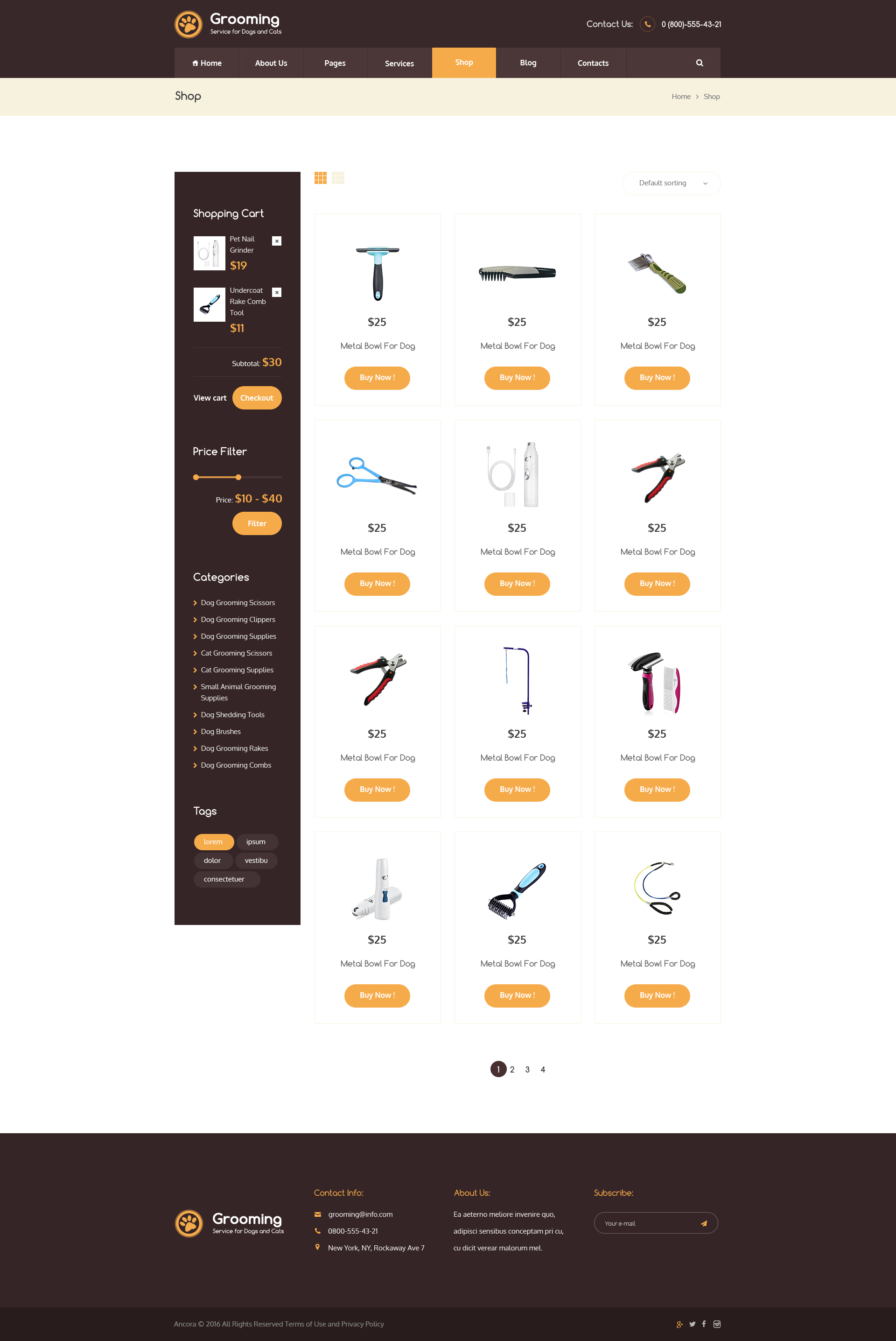The desktop screenshot displays the homepage of a pet grooming e-commerce website. 

In the top left area, slightly towards the center but still on the left side, there's a section likely titled "Grooming for Dogs and Cats." Due to the blurriness, the exact wording is unclear. Below this title, the company’s logo appears as an orange circle featuring a paw print in the center. 

To the immediate right, there's a "Contact Us" section with the phone number 0800-555-4321. This portion of the screen has a dark brown, almost dark maroon background. Directly beneath this header is a navigation menu listing several options: "Home," "About Us," "Pages," "Services," "Shop" (which is currently highlighted in a light orange color), "Blog," "Contacts," and a magnifying glass icon for search functionality. The right side of the menu features a shopping cart icon with several purchasing options.

The main content area sports a white background showcasing featured products. One highlighted item is a metal dog bowl priced at $25. The bowl's image is accompanied by a logo resembling a window scraper. Right beside it, another entry labeled "Metal Bowl for Dog" also priced at $25 showcases a different logo that looks like an ear of corn. Both items include orange pill-shaped "Buy Now" buttons with white font just below their images.

Additionally, underneath the first product image, there’s an item featuring scissors, similarly described as a metal bowl for dogs, priced at $25, with the same "Buy Now" button beneath it. The page generally appears to be a template or placeholder for this pet grooming e-commerce site, featuring repetitive product descriptions and layout elements.